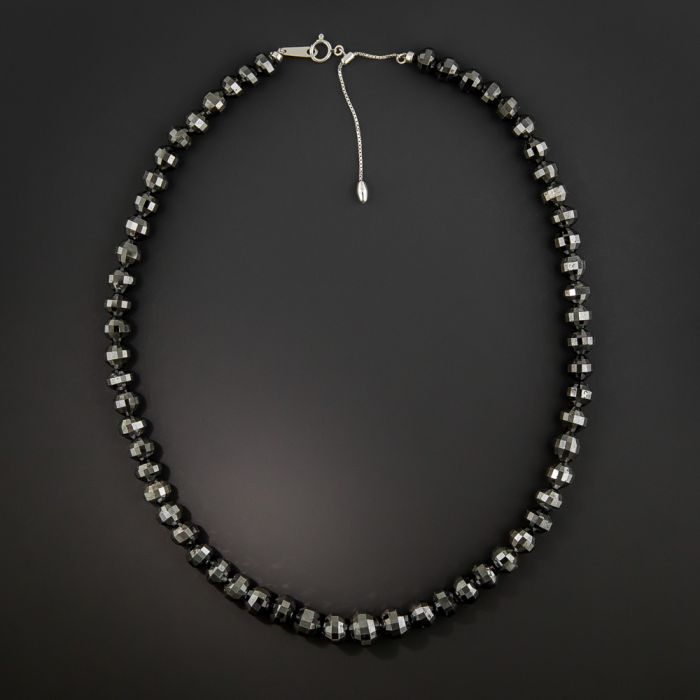This photograph captures a striking beaded necklace set against a black gradient background, enhancing its visibility and detail. The necklace features several 1 1/4 inch black beads, which are slightly sparkly, possibly made of hematite with its typical grayish, shiny tone. These beads are arranged on an adjustable silver chain designed for varying neck sizes. The clasp at the top, consisting of a ring closure and loop, allows for a secure fit. The necklace’s choker style suggests it fits closely around the neck, offering a stylish, elevated look without draping down too far. The thoughtful composition ensures the necklace stands out clearly against the nuanced dark background.